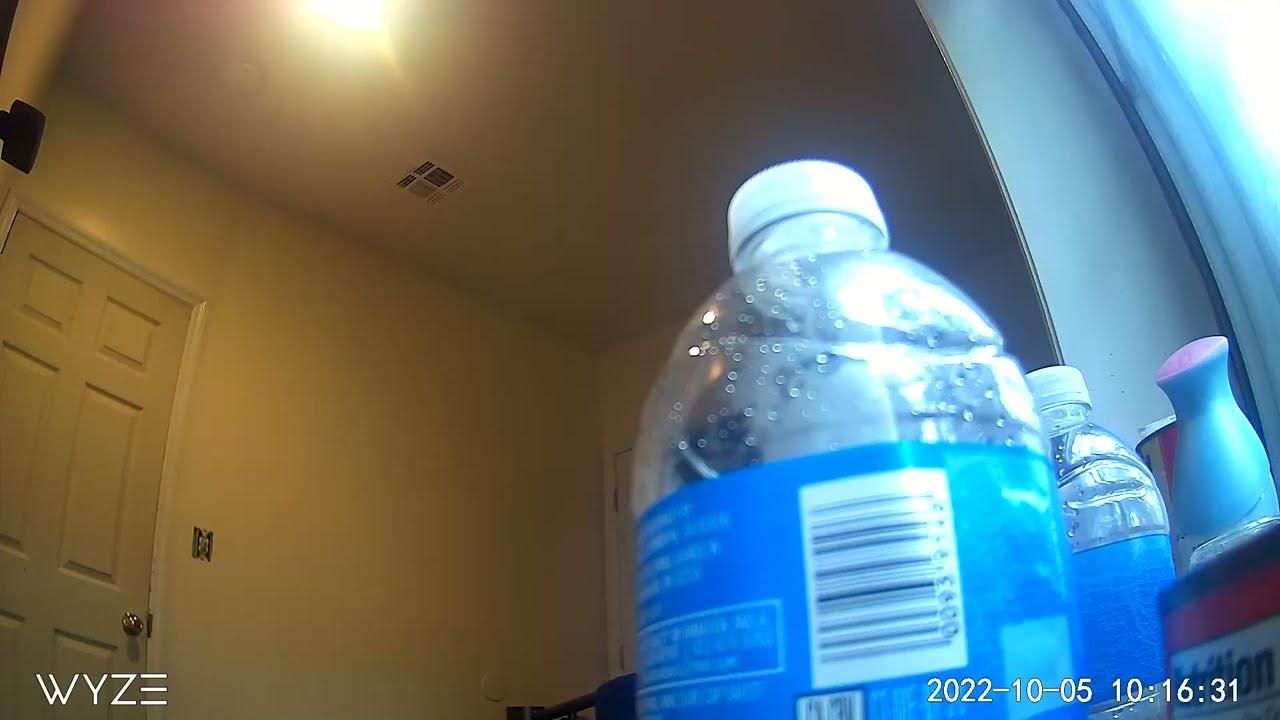This image appears to be security camera footage of a small interior room, captured with a fisheye lens that causes the sides of the image to curve inward slightly. The bottom left corner displays the text "WYZE" in capital letters, indicating the brand of the camera. The date and time stamp "2022-10-05 10:16:31" is visible in the bottom right corner.

The room features light yellow walls and a white ceiling with a bright yellow light shining down. The camera seems to be positioned low, likely on a table or windowsill, giving an upward view of the space. In the foreground, there are two clear plastic water bottles with blue wrappers, condensation visible inside, and a spray bottle that appears to be a Febreze air freshener. One of the water bottles has a visible barcode. These items are situated near a window that allows natural light to enter the room.

In the background, you can see a closed door with a metallic doorknob and an air vent on the ceiling. There is also an electrical outlet or switch without a faceplate visible on one of the walls. The overall impression of the room is utilitarian and unadorned.